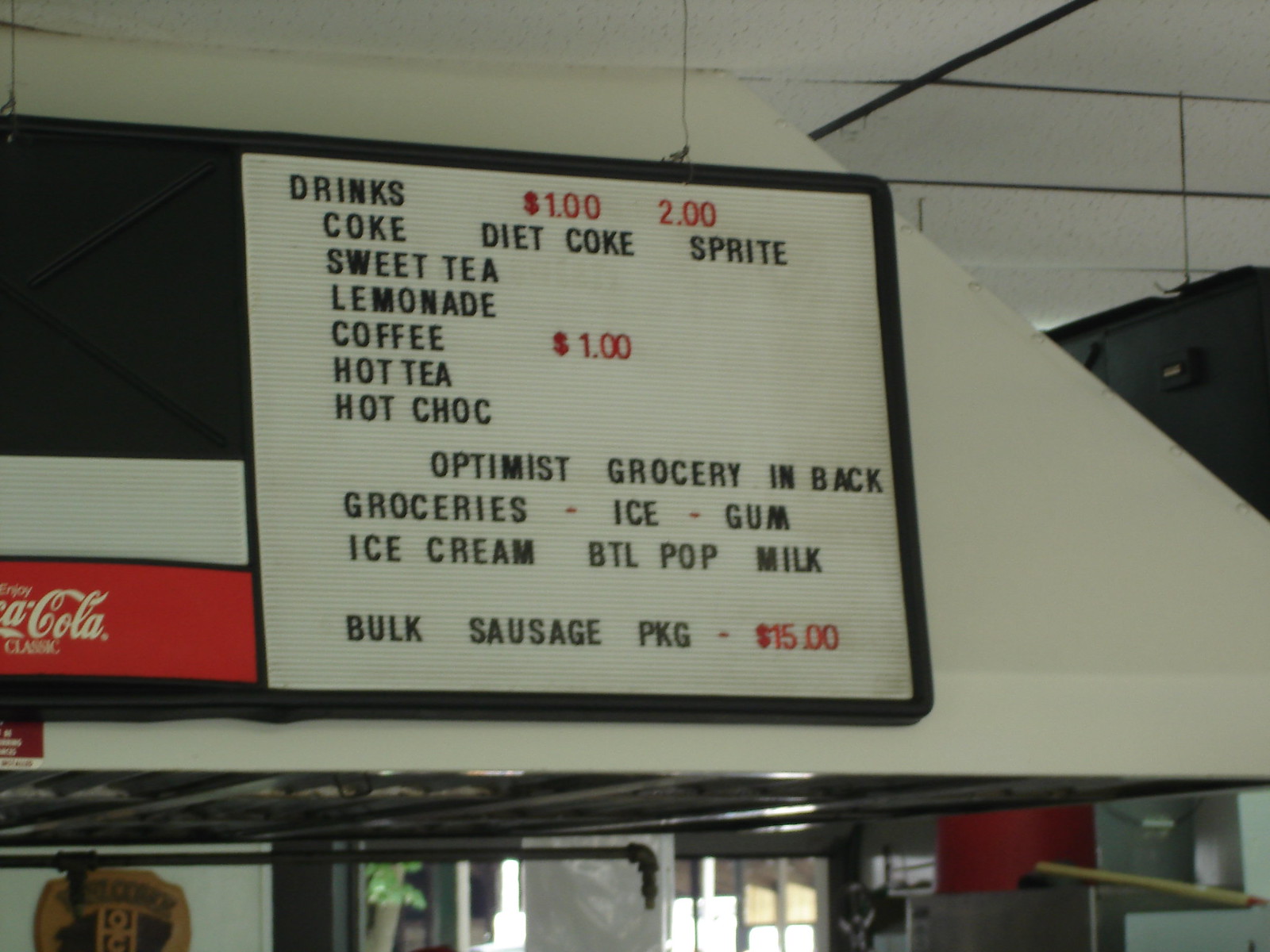The image is a color photograph featuring a menu displayed in either a restaurant or a grocery store. The menu itself is set against a white background and framed with a sleek black border. It is mounted atop an awning-like structure, which appears to be situated above a serving area.

The menu is composed of individual letters and numbers, typical of a customizable sign board. The items listed on the menu are in black text, while the prices are highlighted in red.

At the top, the menu categorizes "Drinks" which includes:

- $1: Coke, Diet Coke, Sprite, Sweet Tea, Lemonade, Coffee
- $2: Hot Tea, Hot Chocolate

Midway down the sign, it states "Optimist Grocery" in bold, followed by a list of available items such as:

- Groceries
- Ice
- Gum
- Ice Cream
- Bottle Pop
- Milk

Towards the bottom, the only prominently priced item is a "Bulk Sausage Package" listed at $15.

The composition of the photograph reveals the setting's ceiling, painted in a clean white hue. To the left of the menu, part of a narrow, rectangular Coca-Cola sign is visible in red and white, adding a touch of classic branding to the scene.